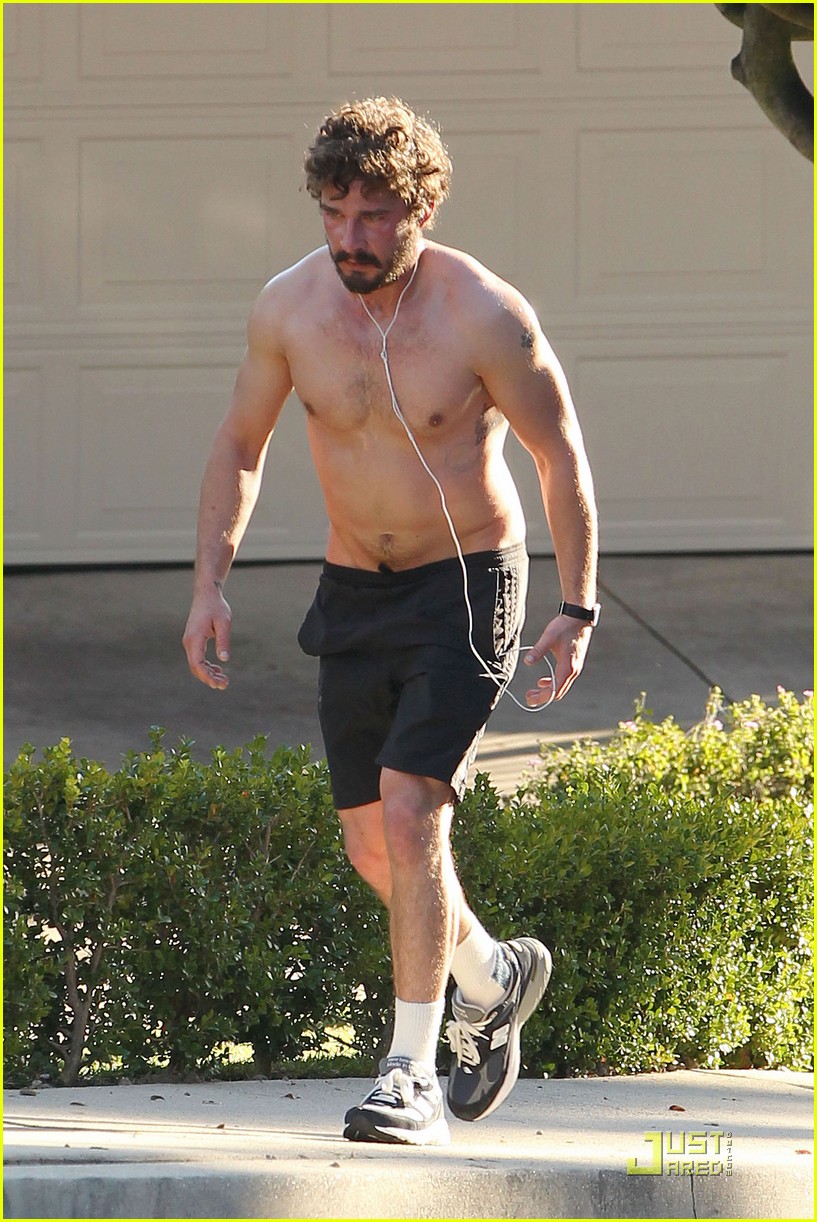The image depicts a shirtless white male with curly brown mid-length hair, a goatee, and a mustache, appearing slightly flushed and sweaty. He is wearing wired white earbuds, black shorts, white socks, black and white sneakers, and a black watch on his left arm. The man, who might be an actor or a celebrity, seems unaware of being photographed, suggesting the picture was taken by paparazzi or a fan. He is walking down a sidewalk, passing by green bushes and hedges that reach up to his knees. Behind the hedges, there is some concrete and a cream-colored garage door, indicating a neighborhood setting. The image includes a small yellow logo in the bottom right corner that reads "Just Jared" alongside the text "dot com."